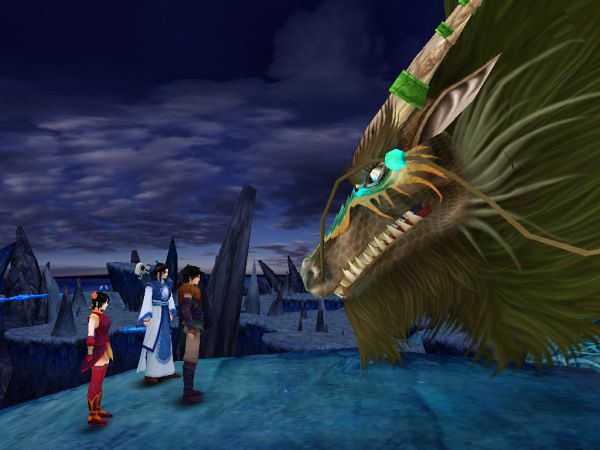This screenshot from an early 2000s-era video game, reminiscent of the PS2 era's characteristic graphics, depicts three characters standing in a dark wasteland beneath a foreboding, dark sky with purple and gray hues. The setting seems laden with jagged stones and gray, black rocks, evoking a desolate mountainous region. At the center-left of the image, the characters are dressed in traditional Chinese clothing, suggestive of a wuxia genre. The first character dons a blue and white robe, the second, a female, wears short red robes over a white shirt, and the third is clad in light brown pants and a brown top. To the right, a massive, mythological Asian dragon with a serpentine body looms menacingly. The dragon, with catfish-like whiskers, green-ringed horns, a green beard, brown gills, and blue and yellow markings around its eyes and snout, snarls at the trio. The scene's overall atmosphere suggests a critical, dark moment in the game's storyline.